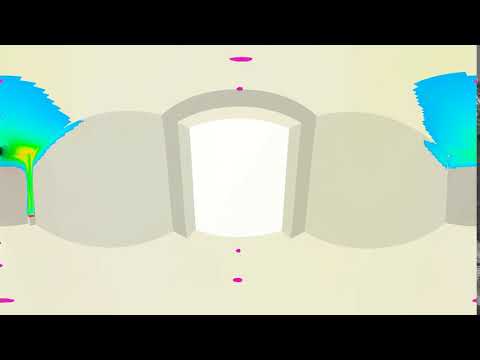The image depicts a 2D, almost cartoon-like low poly scene of a stylized room with a predominantly tan background. The central feature is a bright white arched doorway, outlined by a light gray arch. Adjacent to the doorway, on both the left and right sides, there are gray cylindrical objects or paintings. Beyond these cylinders, there are areas of light blue, possibly representing painted sections or digital anomalies, with the left blue area including a yellow splotch at the top, resembling a plant or tree. The painting also includes splashes of magenta dots distributed throughout — at the very top, center, middle bottom, and the left and right edges. The scene features black lines at the top and bottom, enhancing the cartoonish appearance. The ceiling is white with a distinct red light, contributing to the overall white and gray palette of the room, balanced by the light green accents.